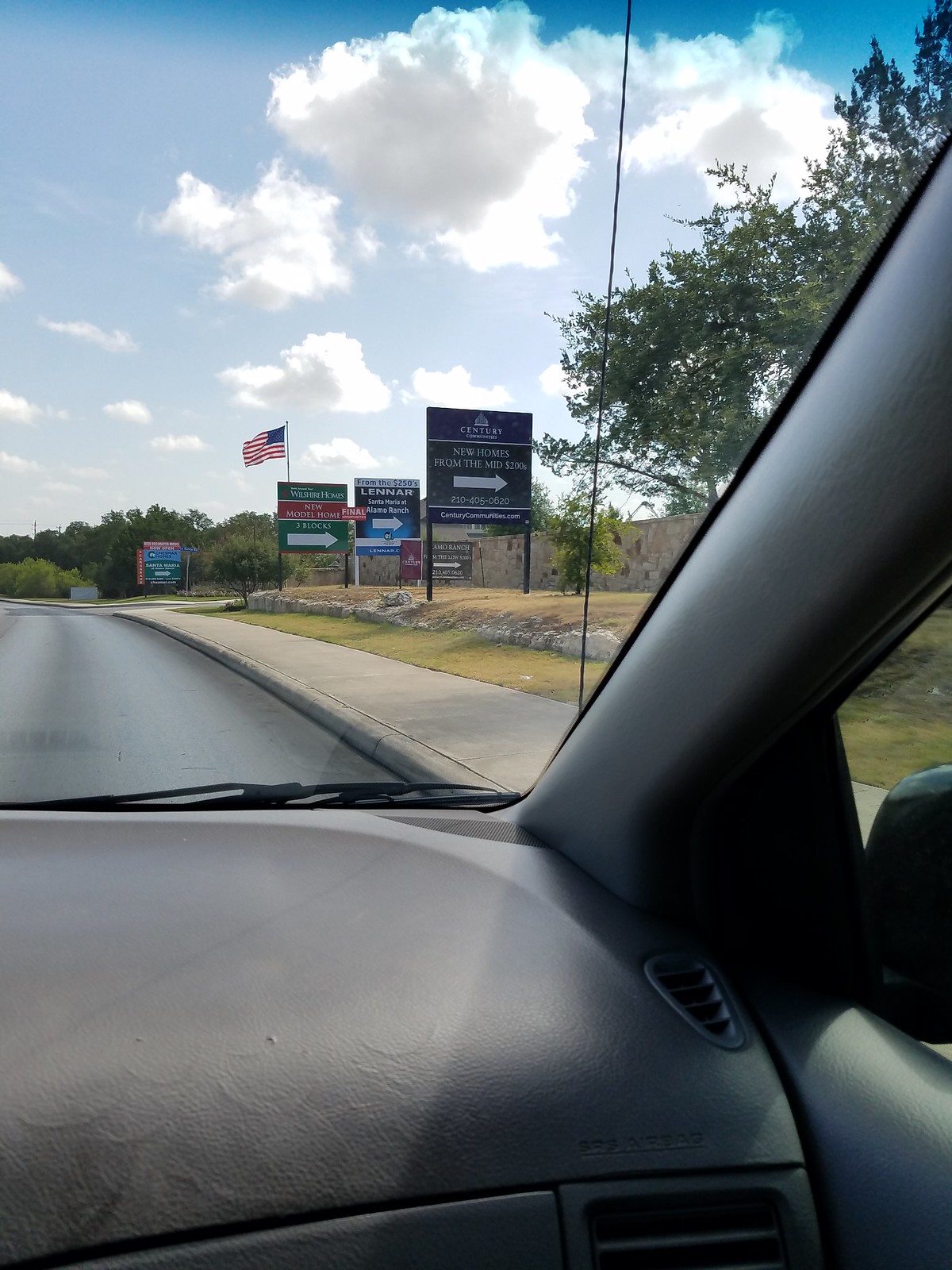A photograph taken from the passenger seat of a car driving on the right-hand side of a US road. The image shows the grey interior of the car, including the dashboard, part of the glovebox, the A pillar, and the wing mirror. Looking out through the windshield, past the antenna, there's a sidewalk and a stretch of lawn on the right side of the road. Several wooden signs are gathered in the distance, all pointing to the right, with at least one reading "New Homes from the mid-7000s" with "Century" at the top. Another sign below that says "Lennar" with similar text, and yet another reads "New Model Homes." An American flag is prominently raised behind the cluster of signs. More signs can be seen farther back, indicating this is a newly developed suburban area. In the distance, there's a bank of trees and a bright blue sky filled with fluffy clouds.